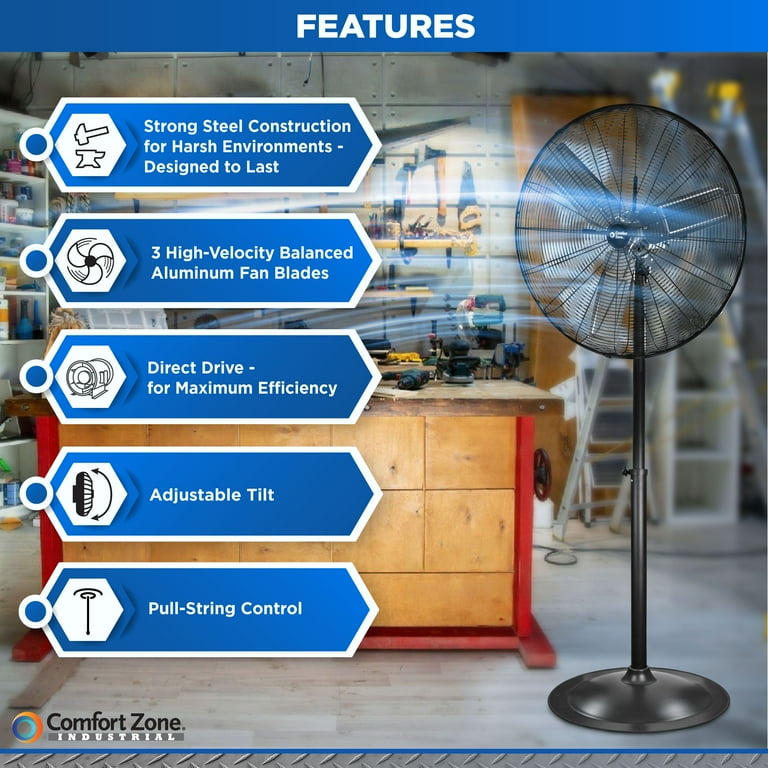This advertisement features a tall, industrial floor fan positioned inside a workroom or garage setting with tools hanging on the walls and a wooden table with power tools nearby. The fan's attributes are highlighted in five blue tags with white trim on the left side of the page, under a blue header that reads "Features" in white text. These features include strong steel construction for harsh environments designed to last, high-velocity balanced aluminum fan blades, direct drive for maximum efficiency, adjustable tilt, and pull-string control. Each tag is accompanied by small icons for visual reference. At the bottom left, the company's logo, a blue and orange circle, is displayed with the text "Comfort Zone Industrial."